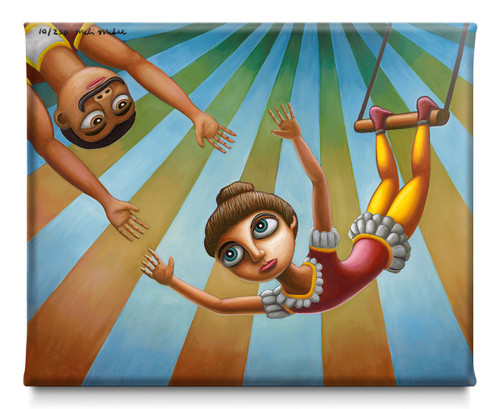The image portrays a vibrant and dynamic scene of two circus trapeze artists suspended in mid-air, reaching out towards each other in a moment of anticipation. On the right side, a woman with black hair styled in a bun is gracefully hanging by her feet from a trapeze swing, her red leotard and shorts contrasting sharply with the backdrop. Her face, positioned lower than her feet, highlights the intensity of the moment as she extends her arms out towards her partner. On the upper left, a mustached man in a colorful costume of white, yellow, and red stretches his arms towards the woman, poised to catch her in mid-swing. The setting is accentuated by the vibrant stripes of the circus tent in the background, alternating in colors including white, yellow, blue, and greenish-blue, creating a lively yet nostalgic atmosphere. The image, reminiscent of a modern painting or computer graphic, is numbered "10 out of 230" and bears the artist’s signature, adding an element of authenticity and exclusivity.